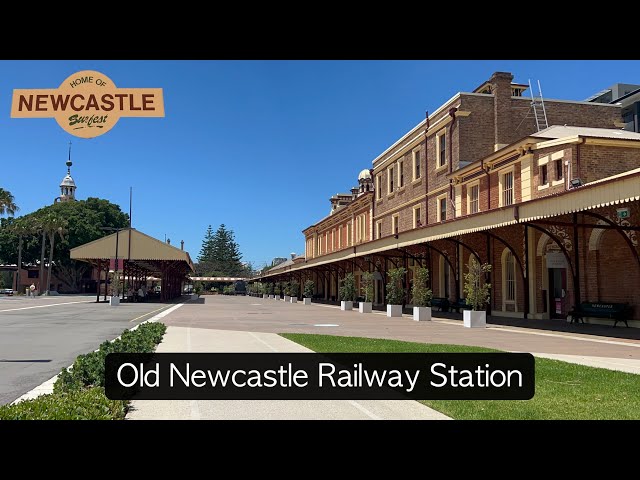The horizontally aligned rectangular image features a picturesque scene dominated by a clear blue sky, bordered by thick black bars at the top and bottom. In the upper left corner, a khaki-colored badge bears the text "Home of Newcastle Sunfest," highlighting a local festival. Below the image, a black rectangle with white text reads "Old Newcastle Railway Station," indicating the location.

The right side of the image showcases a historic brown brick building with arched windows on the first floor and rectangular windows on the subsequent levels. This building is part of the railway station complex, connected by an overhang under which there are benches and white square pots with plants, suggesting a waiting area or ticketing zone. A ladder is visible on the side of the building.

On the left side, a large paved parking area is seen, accentuated by a sidewalk with small shrubs and green grass. Further left, another overhang structure provides shelter and appears to be another waiting area with benches beneath it. Trees and dense foliage frame the background, with a distinctive tower featuring a steeple emerging from the greenery. This detailed scene captures the charm and historical ambiance of the Old Newcastle Railway Station amidst its surrounding environment.